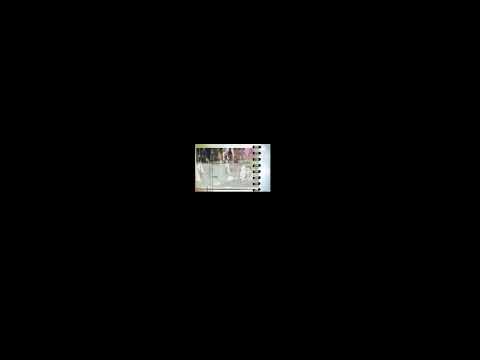The image features a completely black background that fills the entire frame, drawing immediate attention. At the very center of this stark black backdrop is a small, white, rectangular element that resembles a photo album or a stamp. The rectangle is adorned with a series of black, circular details along its right edge, hinting at a spine or a spiral notebook structure. The internal image within the white rectangle is too small and blurry to discern clearly but appears to contain varying shades of pink, green, white, and gray, possibly depicting a head or another unclear object. Despite the ambiguous details, the central focus remains this small, colorful rectangle cocooned in an expansive sea of blackness.